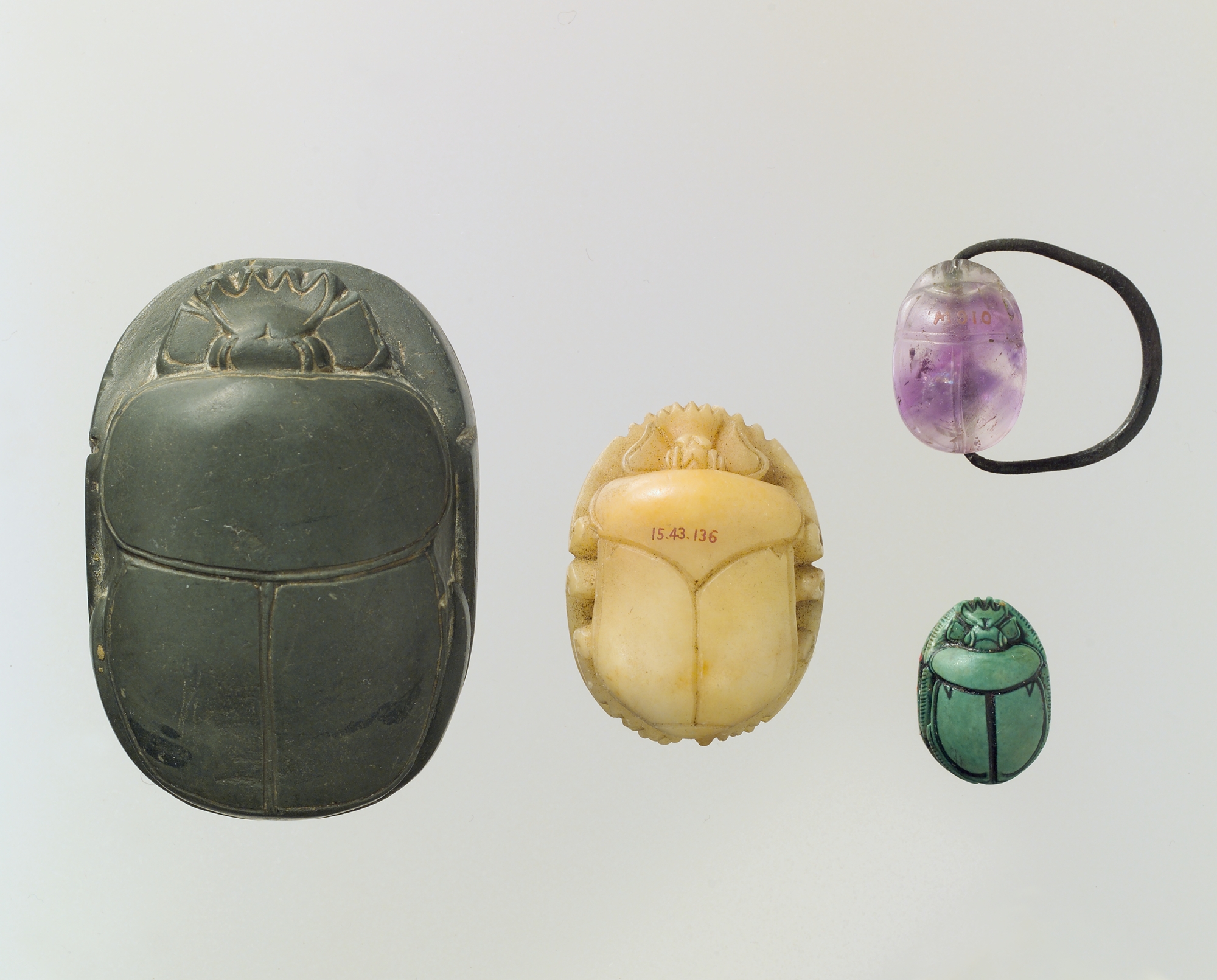The image features a greyish-beigish background showcasing four intricately carved objects that resemble beetle shells, viewed from the top down. The largest object on the left is dark green and has a pattern reminiscent of a turtle shell with additional carvings at the top that look like a webbed foot. The middle object is significantly smaller, about a quarter of the size of the largest, and is a golden-yellow color with the numbers "15.43.136" stamped in red across its surface. To the right are two smaller objects, positioned one above the other but slightly misaligned. The bottom right object is a lighter shade of green and has a distinct face at the top, resembling a small backpack with a gremlin peering out. Above it, the top right object is translucent with a pinkish hue and features a black metal buckle, suggesting it could be attached to a set of keys. The materials appear to be either soap or stone, and despite their mysterious nature, the objects consistently evoke the appearance of beetle shells through their detailed carvings and varying colors.